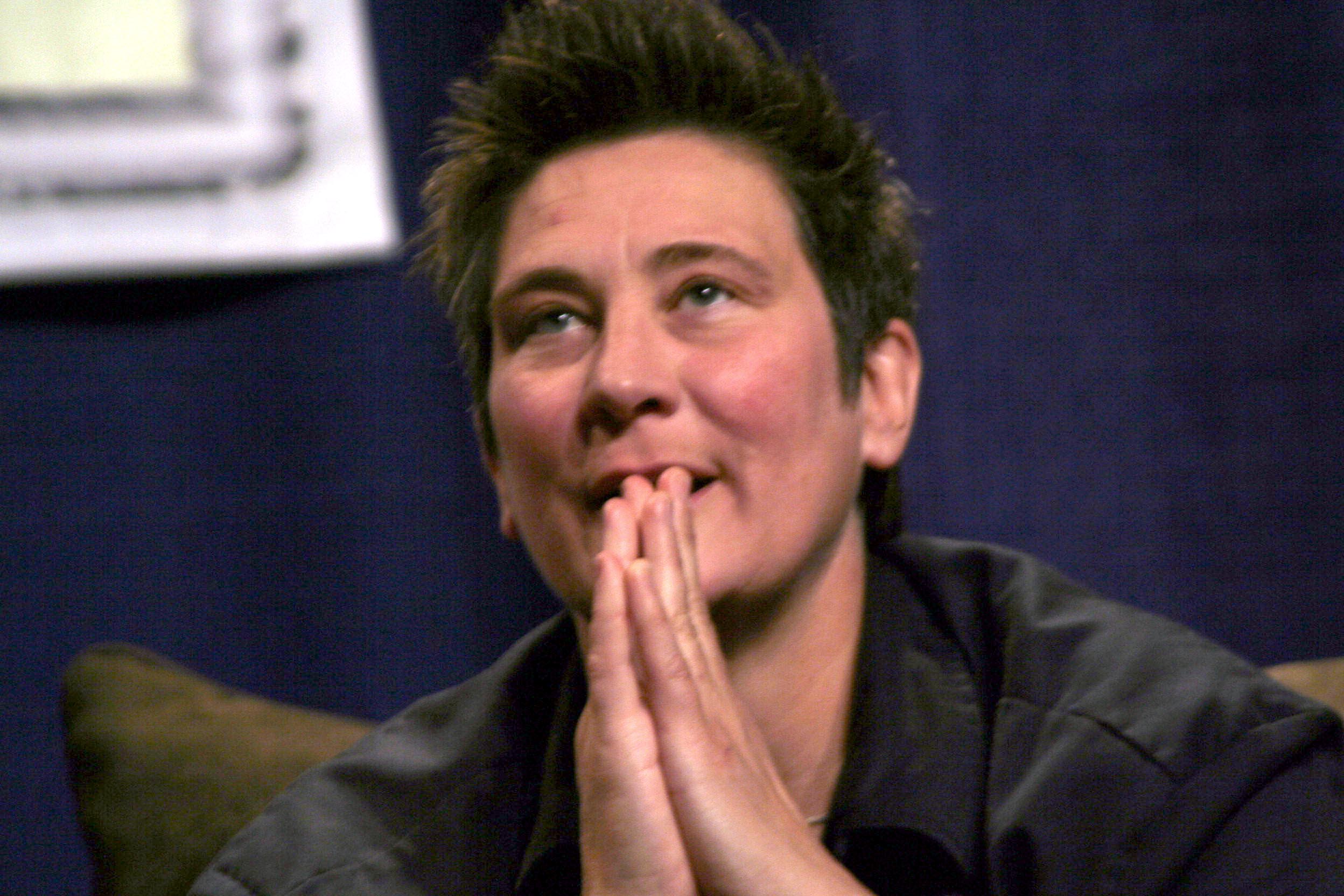The photograph captures K.D. Lang, a woman positioned centrally, seated on a green chair amidst a casual setting, likely during an interview. Her short, spiky dark brown hair complements her attentive gaze directed upwards, revealing thoughtful contemplation. Dressed in a dark, possibly black collared shirt, she appears engaged, with both hands pressed together in a prayer pose in front of her mouth, suggesting she is about to speak on a matter of significance. The setting includes a beige, green, brown, black, white, olive green, and navy color palette, with a medium to dark blue or purple backdrop. The background also features a white-framed corner, adding to the setting's informal yet deliberate atmosphere.